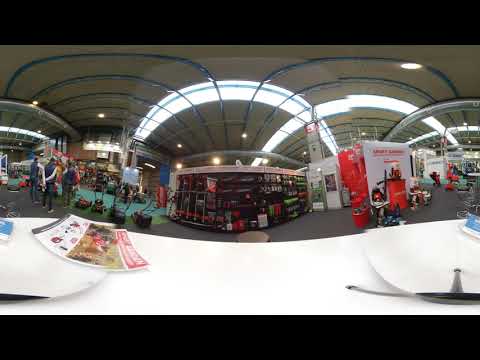The image, captured through a fisheye or VR camera lens, showcases a large, indoor space that includes different stores. The distortion from the lens makes the scene appear curved, giving a panoramic feel. Prominently on the left side, there is a row of lawnmowers positioned on a green surface, with several people milling around nearby, indicating a busy, bustling atmosphere. In the foreground, a counter is visible with flyers on top, some resting on white, disc-shaped objects with blue leaflets. 

Central to the image, there’s a display case with a white strip at the top, containing various items inside containers. Further drawing attention upwards, the ceiling features a significant architectural element: a lit, half-circle at the top center with a thin teal line and blue arches radiating from the middle to the sides of the room, suggesting a modern, structured ceiling design. The right side of the image shows a white and red box positioned on the floor, enhancing the visual complexity of this busy indoor scene.